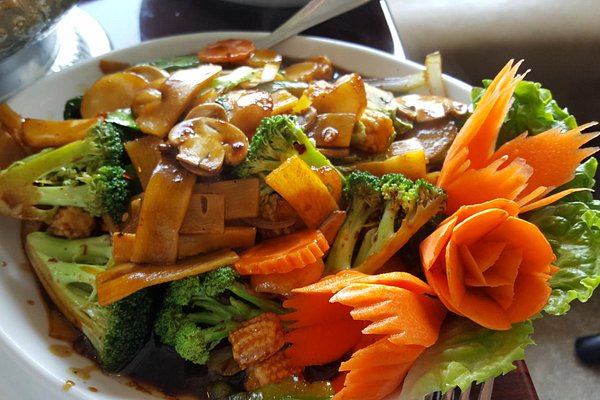This is a detailed color photograph in landscape orientation, showcasing a beautifully arranged, oval white platter of Chinese cuisine. The dish is visually inviting with a mix of vegetables and wide noodles, all covered in a rich brown sauce. Predominantly on the left side, there are finely sliced potatoes or a similar starchy vegetable, interspersed with savory mushrooms, and bits of broccoli. The broccoli is mainly centered at the bottom, accompanied by baby corn underneath. To the right, the platter features an artistic garnish: a rose meticulously carved from a carrot, flanked by decorative carrot leaves. Below this intricate carrot flower lay one or two large lettuce leaves, adding a leafy green contrast to the colorful vegetables. At the top middle of the image rests a silver utensil, indicating the meal is ready to be enjoyed. The background subtly fades, keeping the focus on the vibrant and detailed presentation of the main dish.